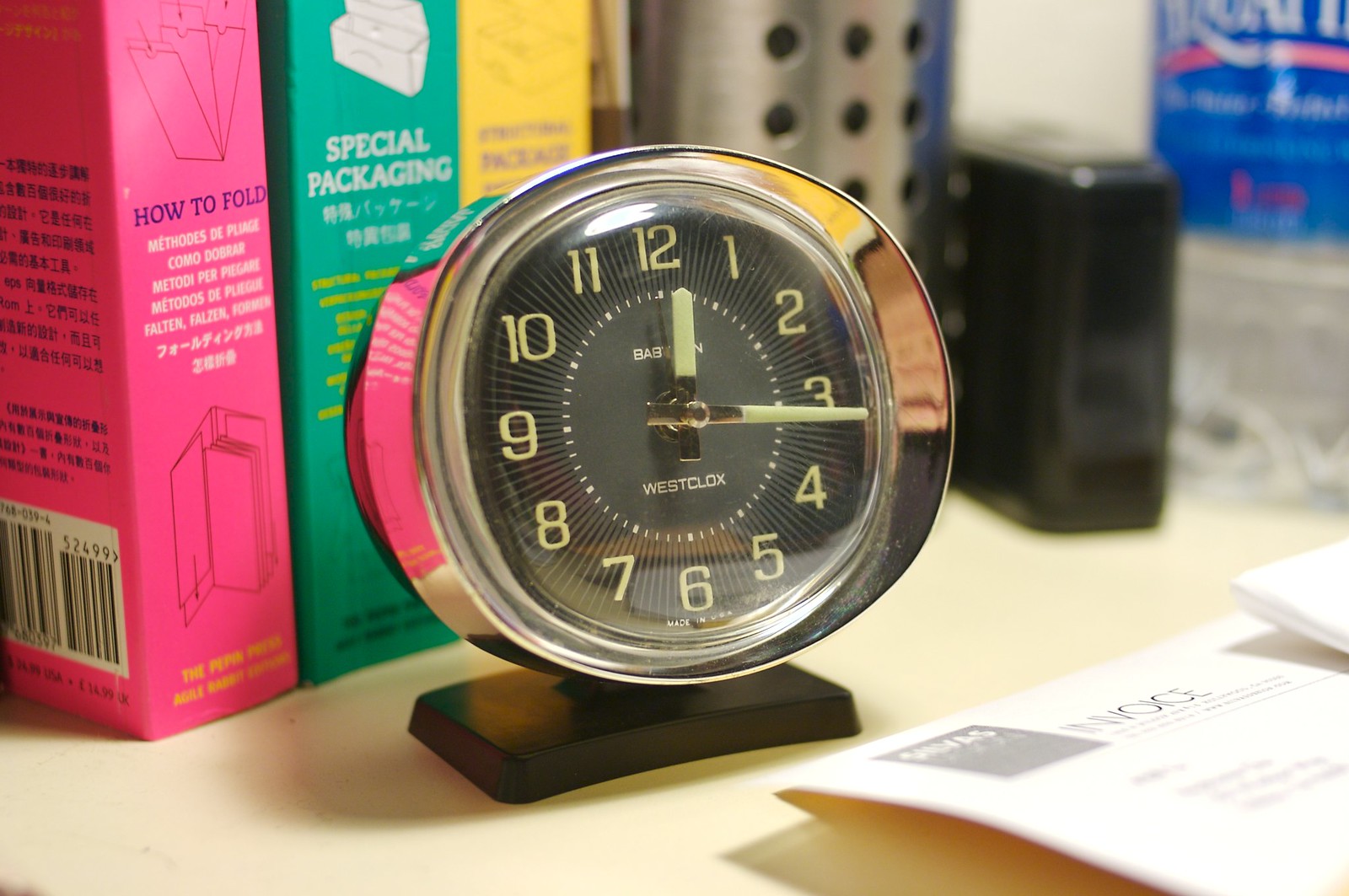This vintage alarm clock, unmistakably nostalgic, sits elegantly on a dark-colored, flat, squarish base. Encased in a chrome circular frame, the clock emanates an old-fashioned charm. The face of the clock features the brand name "Westclox," meticulously spelled out as W-E-S-T-C-L-O-X, and is adorned with luminescent dots that likely allow it to glow softly in the dark. The numbers on its face are arranged traditionally, starting from 12 at the top and proceeding clockwise. The clock finds its home on a well-used desk cluttered with everyday items, including a pencil holder, a bottle of water, and a pencil sharpener, adding to the scene's lived-in appeal.